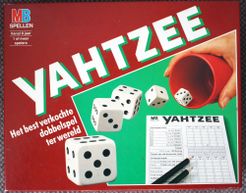The image is a slightly blurry, small rectangular photograph, likely measuring around an inch high by an inch and a quarter wide, capturing the top of an older Yahtzee game box. Predominantly featuring a red background, the upper left corner displays the letters "M" in red and "B" in blue, hinting at the Milton Bradley brand. The word "Yahtzee" is prominently written in large white letters with a subtle green outline, placed diagonally from the bottom left to the top right. Below the title, in smaller white text, are some indecipherable words in German or Dutch, suggesting it's a foreign version of the game.

In the lower section of the box, there is an illustration set against a green backdrop depicting a hand emerging from the right, holding a red plastic cup with dice tumbling out. The visible dice show the numbers six, two, and four, with the remainder still in motion. Below this, a Yahtzee scorecard and two black pencils are arranged, emphasizing the gameplay aspect.